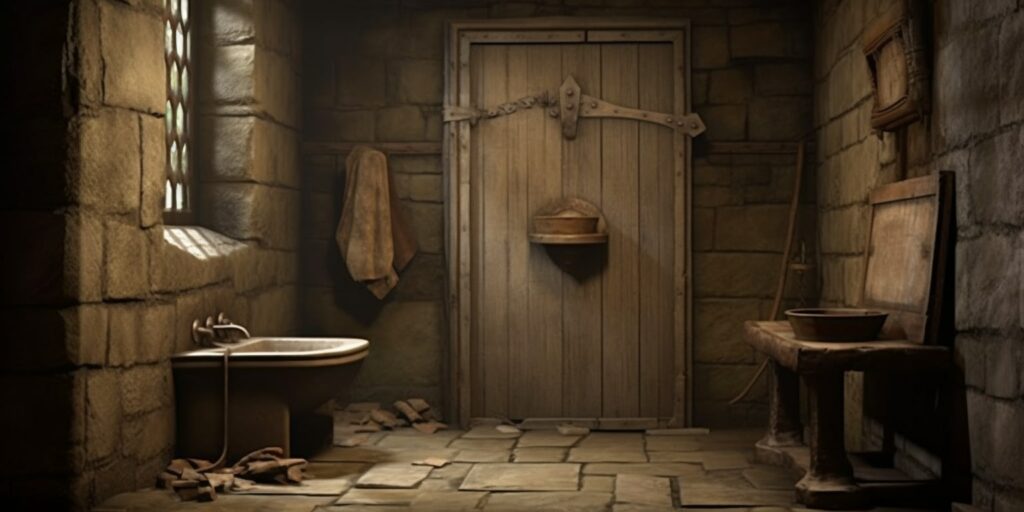This computer-generated image depicts the interior of a small, dimly-lit dungeon bathroom, seemingly located in a castle or medieval structure. The room is constructed with large, grayish-brown stone blocks and features a window with circular holes and a honeycomb pattern, allowing minimal light to penetrate. The window is framed in brown wood. The floor is made of stone tiles that match the walls.

The rustic wooden door, which has a dark, lightish-brown hue, is reinforced with metal braces and rivets and features a large, sturdy lock at the top. Inside the dungeon-like bathroom, a white ceramic sink with multiple faucets and handles stands out against the stone wall. Adjacent to the sink is a primitive toilet consisting of a wooden seat positioned over a bucket.

Additional details include a light brown towel hanging on a rack beside the door, a wooden shelf on the right, and a wooden bowl of the same color as the walls. Scattered on the ground are brown leather straps, and a wooden pole resembling a broom is placed in the back corner. Overall, the scene conveys a stark, unwelcoming atmosphere typical of medieval dungeon settings.